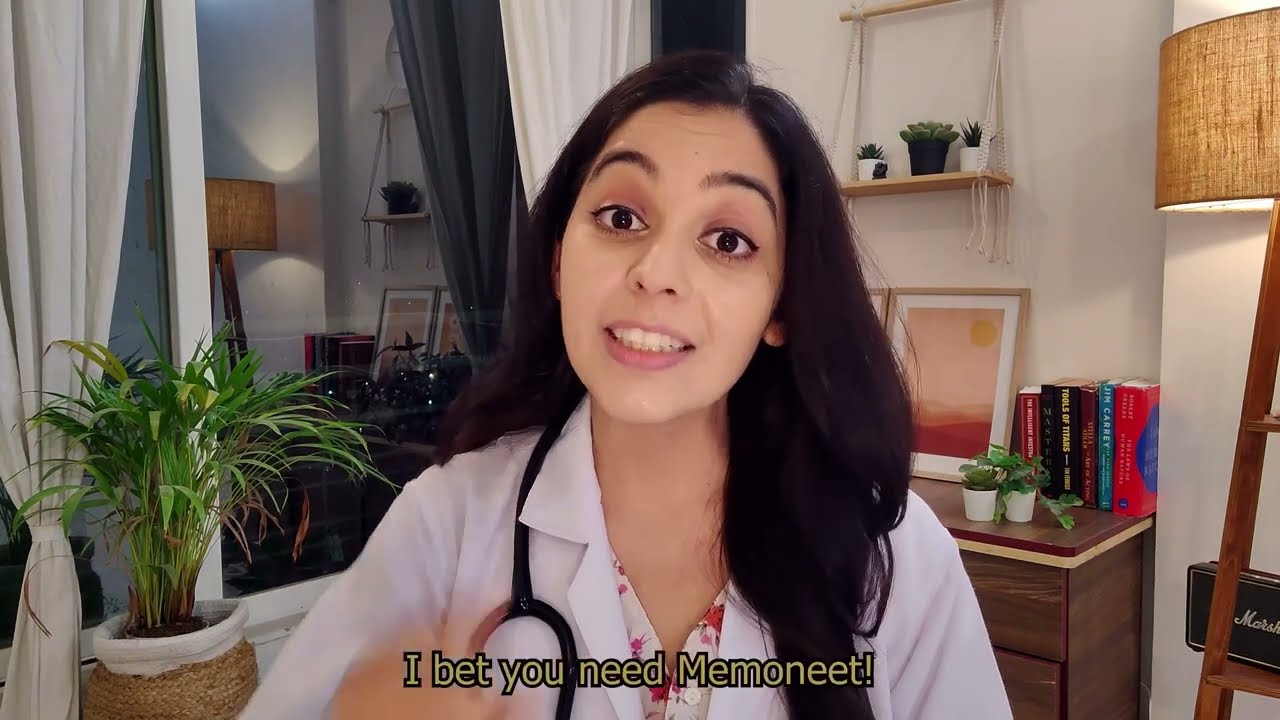In this detailed photograph set in what appears to be a medical office, a young woman with long black hair, black eyebrows, and black eyes is looking directly at the camera with a slight smile. She is dressed in a doctor's white coat with a black stethoscope around her neck, suggesting she is a medical professional. The room features a variety of elements: in the foreground to the bottom left, there's a green potted plant in a wicker basket. In the background, the right side reveals a short end table adorned with books, small plants, and picture frames. Adjacent to the table stands a brown floor lamp. The top right corner also includes a beige shelf holding more small plants, adding to the room's relaxed atmosphere. A window with long white curtains tied to the side allows light to fill the room, and its reflective surface shows the rest of the room. Prominently, at the bottom center of the image, a yellow font with black outline reads, "I bet you need Miminette." Overall, the photograph captures a calm and inviting medical setting with a harmonious blend of colors such as white, gray, green, brown, black, tan, and red.